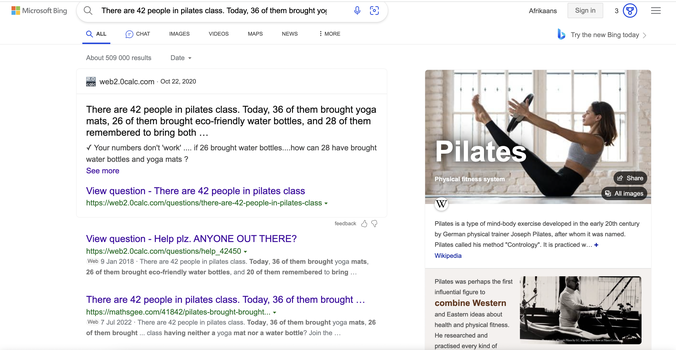A detailed and cleaned-up caption for the described image would be:

"A screenshot of a Microsoft Bing web search engine result displaying a partially visible query: 'There are 42 people in Pilates class, today 36 of them brought yoga mats, 26 of them brought eco-friendly water bottles, and 28 of them remember to bring both,' with the rest of the question truncated. The interface language is selected as Afrikaans, and there is no user signed into any account, indicated by the available 'Sign in' button in the upper right corner. The top search result offers a link to view the complete question, suggesting it might be a homework-related query. In the right panel, a stock photo of a woman holding a Pilates pose is visible, accompanied by information sourced from Wikipedia."